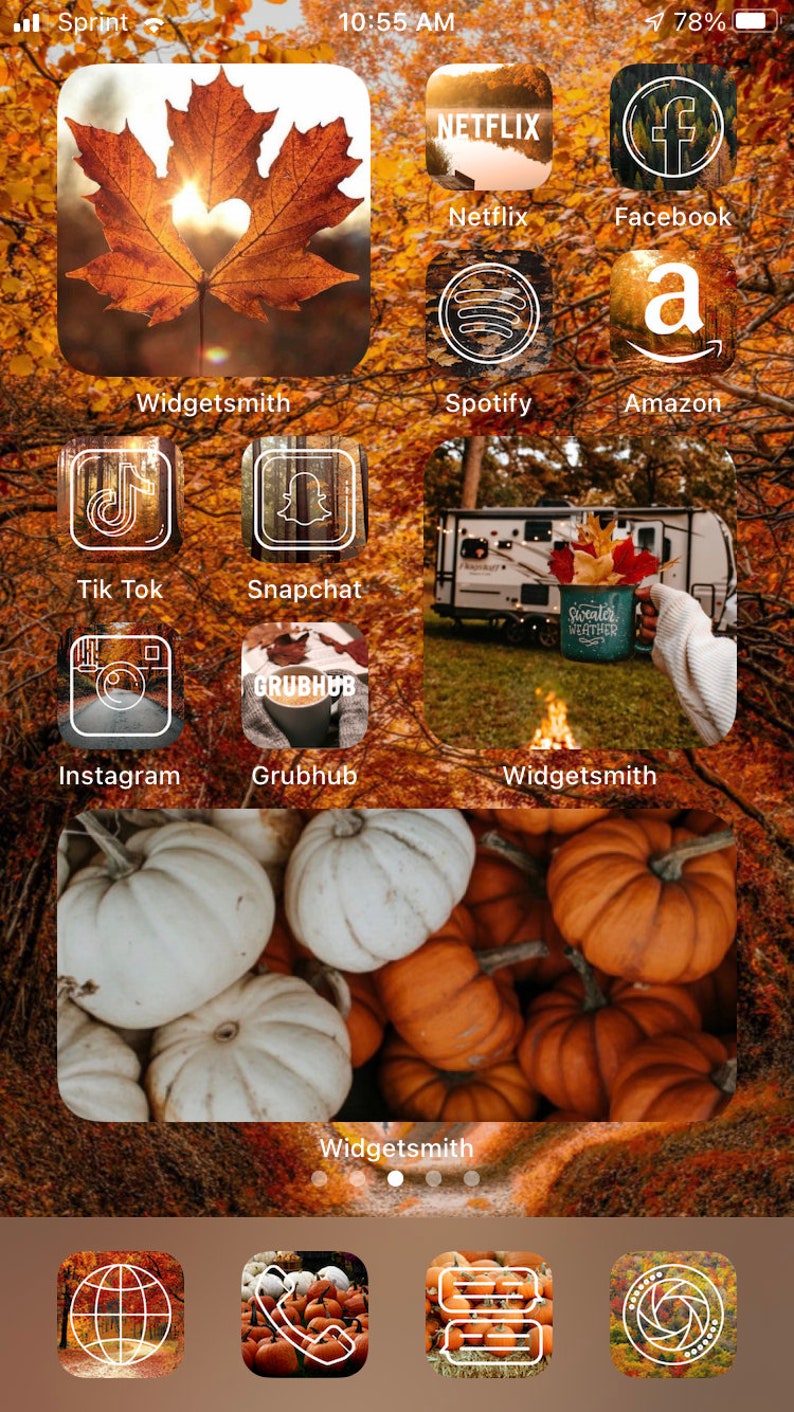This is a screenshot from an Apple device, likely a tablet or phone, running a Mac operating system. The status bar at the top displays several indicators: three bars representing the cellular network strength with the carrier labeled "Sprint," a Wi-Fi signal strength icon with two bars, the time "10:55 a.m.," and a battery level at 78%.

Below the status bar, the home screen showcases various app icons and widgets amidst an autumn-themed background featuring autumn leaves and pumpkins. Prominently, there are multiple icons labeled "Widget Smith," possibly indicating customized folders. One such folder has an icon of a leaf with a heart, resembling a fig or oak leaf.

The app icons displayed include popular platforms like Netflix, Facebook, Spotify, Amazon, TikTok, Snapchat, Instagram, and Grubhub, alongside additional "Widget Smith" folders.

At the bottom of the screen are four main icons: 
1. An image of trees, likely linked to a gallery or nature-related app.
2. A call button, featuring pumpkins which contributes to the autumnal aesthetic.
3. A text messaging icon, which also incorporates pumpkin imagery in the background.
4. A camera icon, assumed to be for accessing the device's camera.

Overall, the screenshot highlights a richly themed autumn interface with a focus on fall aesthetics and popular social and utility apps.